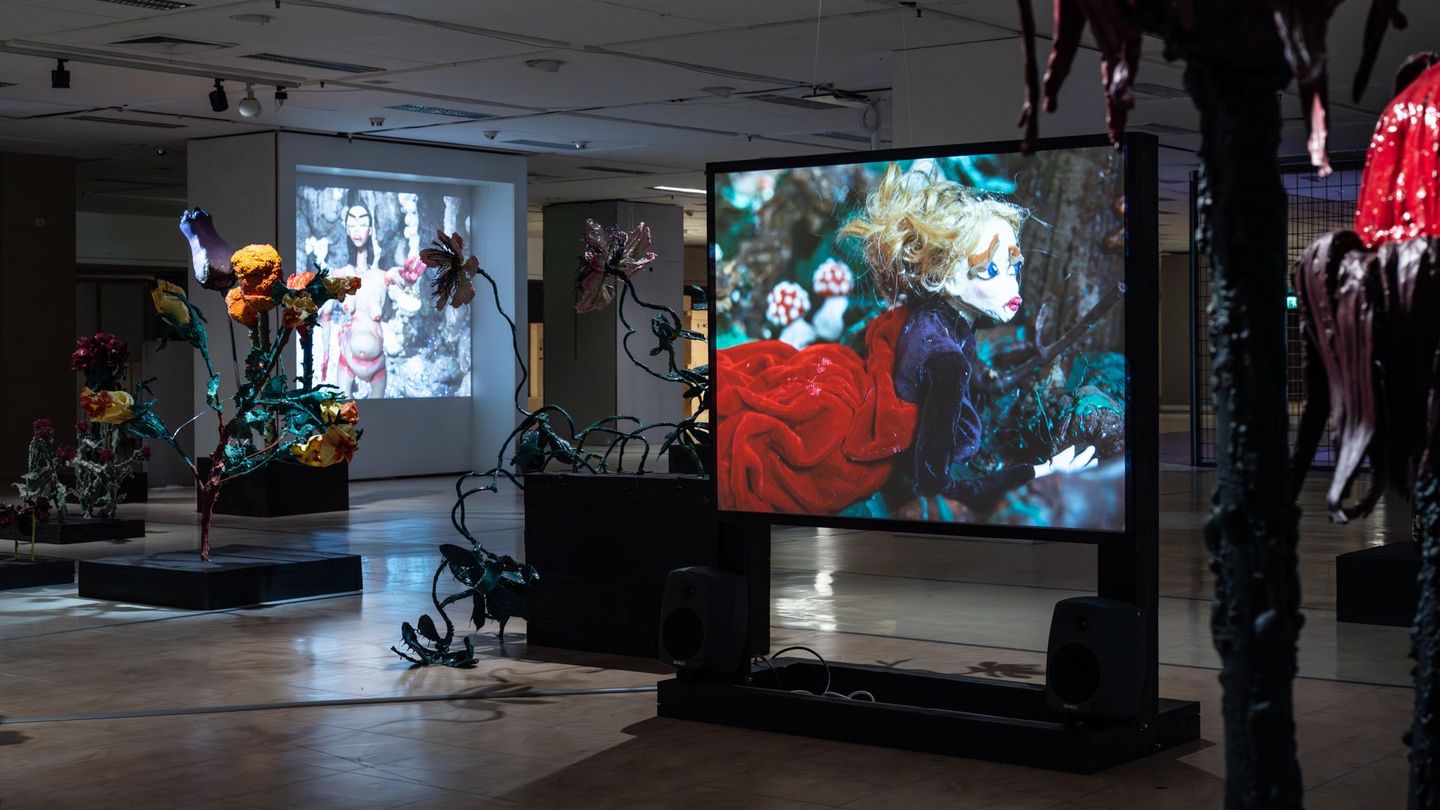The photograph captures a detailed view of an intricate art exhibit set in a large, open, and dimly lit showroom with a low, white ceiling and reflective, gray linoleum flooring. The space features a variety of installations and screens displaying artistic images. On the right forefront, there's a prominent screen displaying a cartoon-like lady dressed in an elaborate black velvet and red gown. To the far left, another screen showcases a character that appears to be nude. The center of the room hosts a large, brightly lit display of a colorful figure resembling a clay-molded person with blonde hair, adorned in vivid hues of red and green. Spanning from the left to the right, the exhibit features an array of sculpted plants and flowers, crafted to look like fantastical creatures, showcasing colors such as purple, yellow, and orange. Additional dark wire sculptures are scattered throughout, further enriching the eclectic and vibrant atmosphere of the gallery-like space.